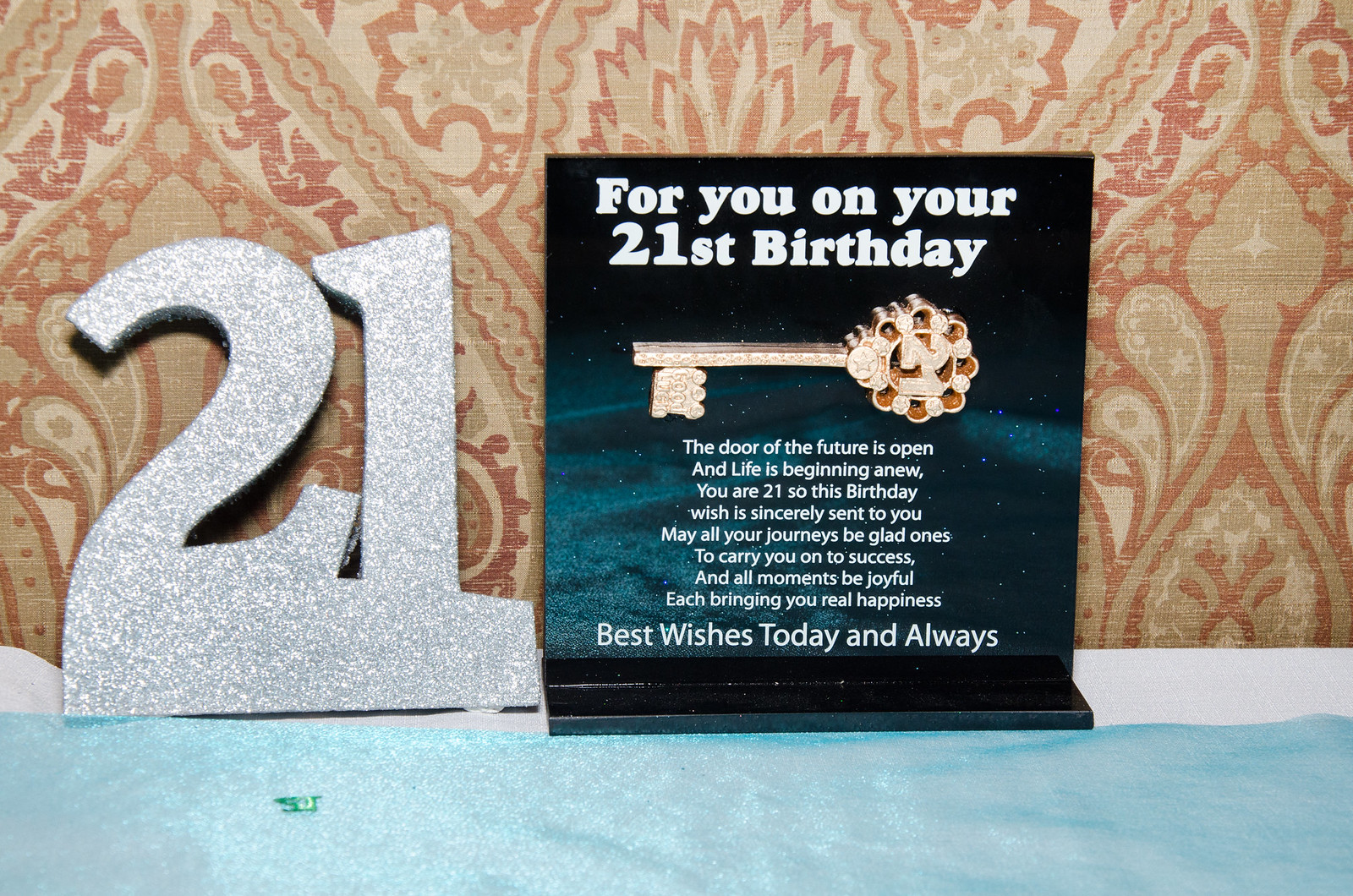This color photograph captures a detailed birthday display for a 21-year-old. On the right, there is a professionally crafted, black advertising sign adorned with a starlight background. In white text at the top, it reads, "For you on your 21st birthday," featuring a three-dimensional golden key graphic. The sign includes an elaborate birthday message: "The door of the future is open, and life is beginning anew. You are 21, so this birthday wish is sincerely sent to you. May all your journeys be glad ones, to carry you on to success, and all moments be joyful, each bringing you real happiness. Best wishes today and always." This sign rests on a blue area that appears to be tissue paper or a similar material. To the left of the sign, a cardboard or Styrofoam cutout of the numerals "21" is displayed in a silver glitter color. Both the sign and the numerals are set against a patterned wallpaper with red, beige, and brown hues, creating a festive and heartfelt birthday tribute. The entire setup sits atop a white table.